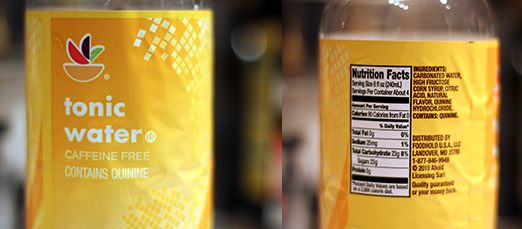This narrow, horizontal image comprises two side-by-side smaller images: the front and back views of a tonic water bottle. The left image highlights the front label, which features a vibrant yellow background with an orange rectangular section adorned with white diamond-shaped bubbles in the upper right-hand corner. Within the orange area, a white semicircle sits at the bottom, from which three slice-shaped objects in red, black, and green rise, resembling citrus wedges. The label also includes inscriptions in white letters that read: "Tonic Water," "Caffeine-Free," and "Contains Quinine."

The right image displays the back of the same bottle, with a predominantly yellow background. Centered is a horizontal nutrition facts label in white, detailing the serving size, fats, sodium, and carbohydrates in black text. Adjacent to the nutrition label, the ingredients and distribution information are printed in brown. It states that the product is "Distributed by Food Hold USA, Landover, Maryland."